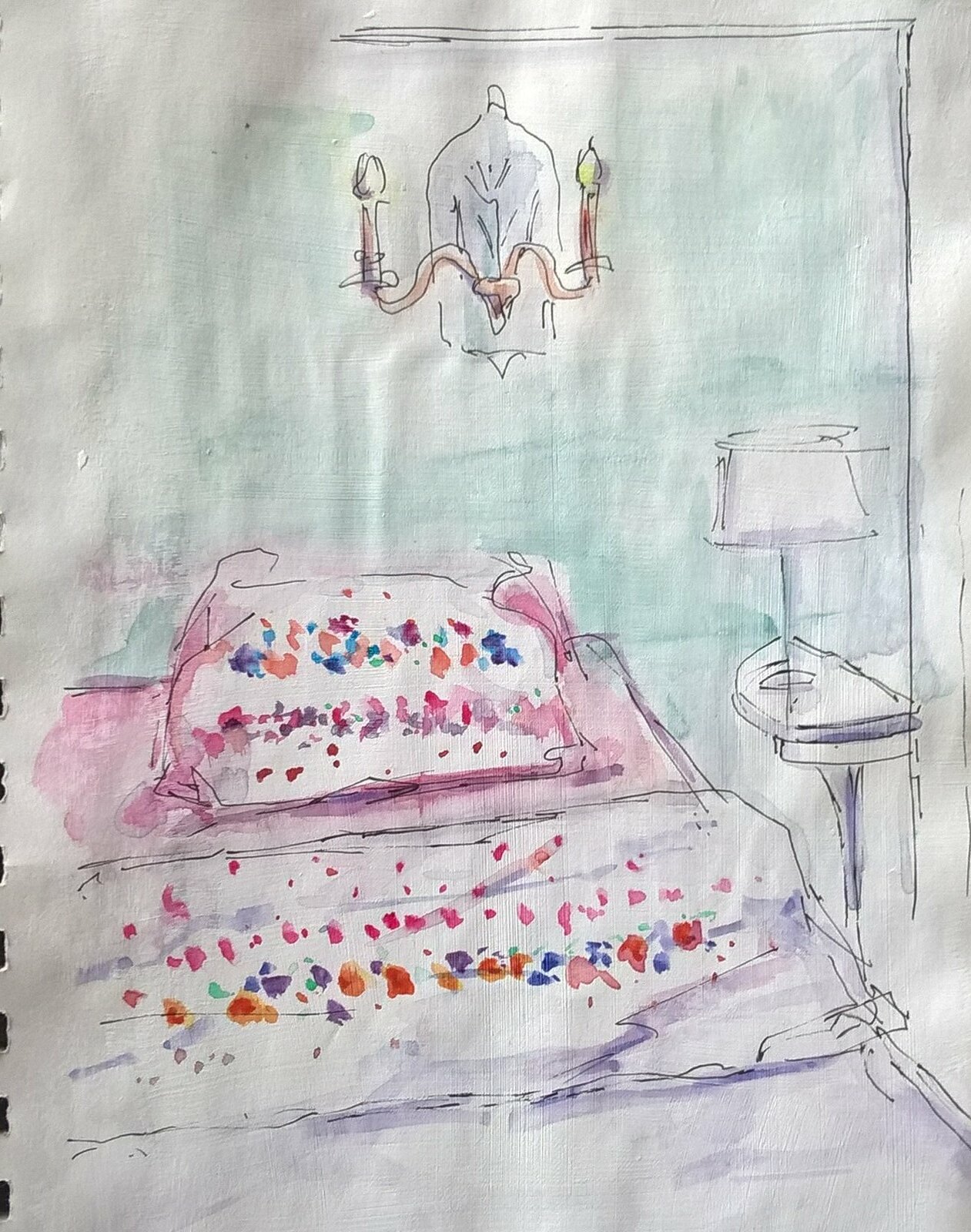A detailed pen and ink with watercolor sketch captures an intimate living area that could double as a sleeping space. Central to the scene is a piece of furniture that ambiguously serves as a bed or couch. The comforter, partially turned over, reveals a floral design edging, depicted with delicate watercolor strokes. Resting atop the furniture is a pillow patterned with colorful specks and floral motifs, suggesting a homey and inviting atmosphere.

Adjacent to this piece of furniture stands a narrow-based night table adorned with a stylish, single-stemmed table lamp. Above, affixed to the wall, is an intricately outlined candelabra, filled in with soft watercolor hues. The background features detailed edging in pen and ink, adding a sense of depth and structure to the corner of the room.

The overall composition adeptly blends the two mediums, creating a cozy and aesthetically pleasing representation of either a serene bed with a turned-over comforter, or a comfy couch adorned with a decorative pillow. The sketch is an exquisite interplay of detailed linework and vibrant watercolor, capturing the essence of a sophisticated yet cozy interior.